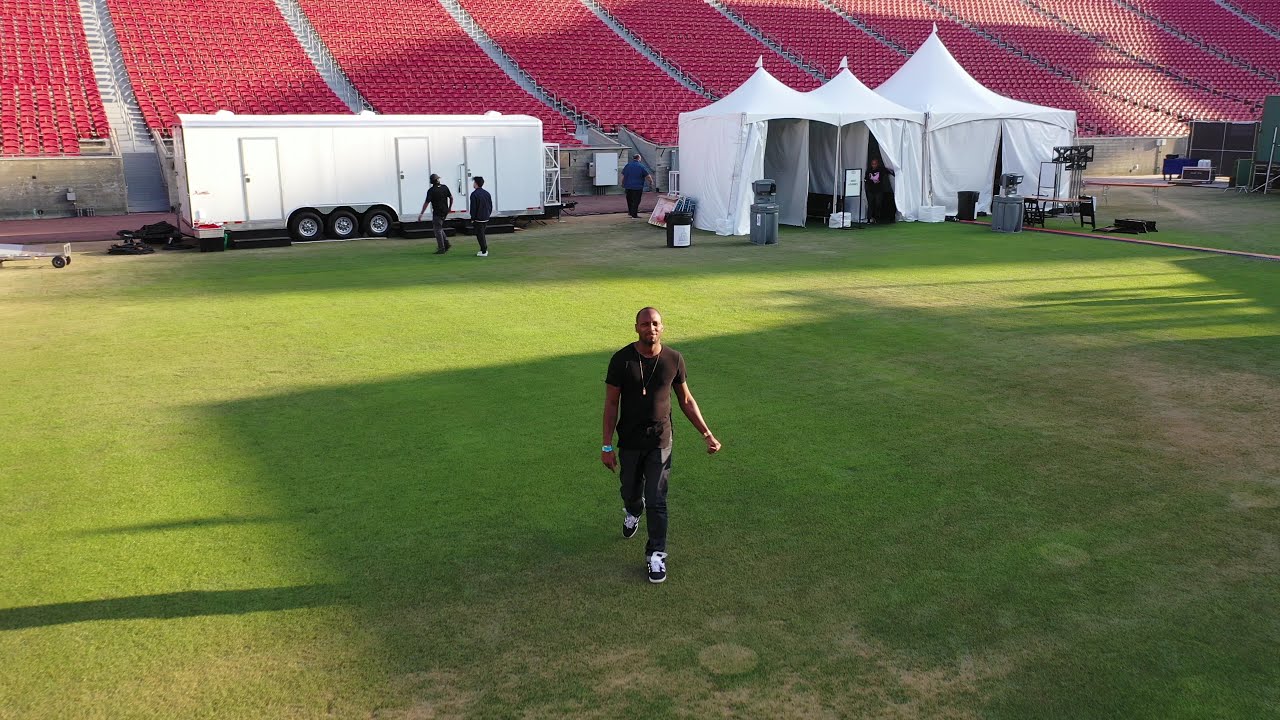This image captures a vibrant scene inside a sports stadium, possibly intended for a football game or a concert setup. Dominating the image is a grass field, patchy with brown spots and basking in the summer sun. Stadium seats are visible in the background, all painted a vivid red, with white railings segmenting the sections. On the left side of the image, a white three-wheeled trailer is parked, near which two men dressed in black are conversing, their attention directed to the left. To the right, multiple white tents are set up along the edge of the field, suggesting preparations for an event, possibly involving directors or catering services.

In the middle bottom part of the image, a man wearing a black t-shirt, black pants, and black sneakers with white soles walks towards the camera, a green wristband visible on his right wrist and a necklace hanging around his neck. Another person, dressed in a blue shirt and black pants, is walking towards the field between the trailer and the tents, while a fourth individual is seen pulling back a curtain on one of the tents. Shadows cast by the upper seating or perhaps a scoreboard add a dramatic element to the scene, reinforcing the impression of an active, bustling environment within this large stadium.